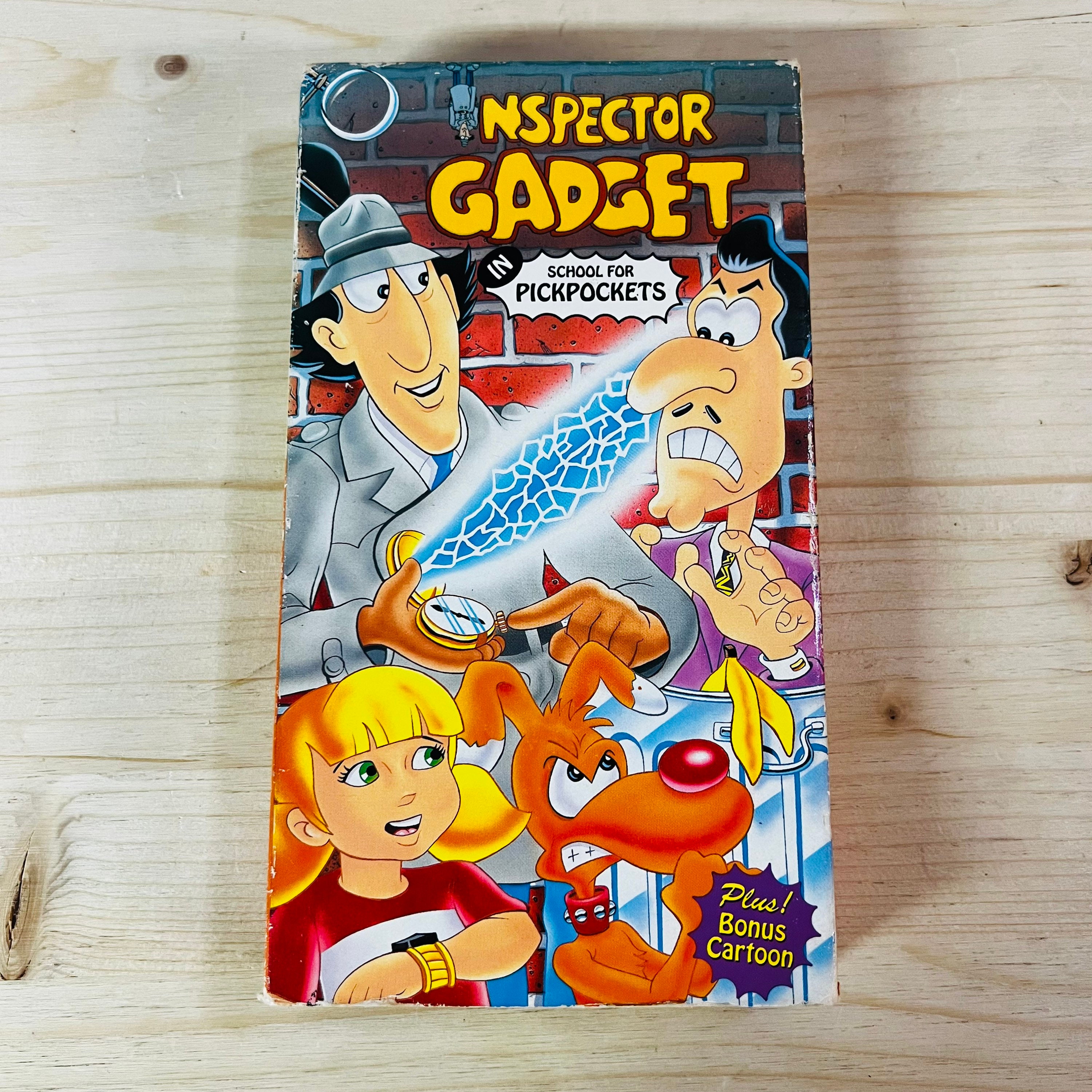The image depicts a vintage VHS tape box of the cartoon "Inspector Gadget," set against a background of light blonde wooden planks. The tape box's cover prominently features the title "Inspector Gadget" in yellow at the top, followed by the subtitle "in School for Pickpockets." Central to the artwork is Inspector Gadget himself, clad in his grey detective hat, grey suit coat, white shirt, and blue tie. He sports a long face with prominent big eyes and a nose, setting his serious yet curious expression. Inspector Gadget is seen facing a scowling villain, who has a pronounced nose, dark hair, a deep scowl, and is emerging from a silver trash can adorned with a banana peel on its rim. This antagonist is dressed in a purple jacket, white shirt, and a yellow and black tie. Below them, on the left side, stands Penny, the young girl known for her distinctive blonde pigtails and red-and-white t-shirt, smiling up towards the action above. Next to her, on the right, is Brain the dog, characterized by his orange fur, red nose, and angry expression, also looking up at the villain. At the bottom of the cover, the text "plus bonus cartoon" is displayed, promising additional content.